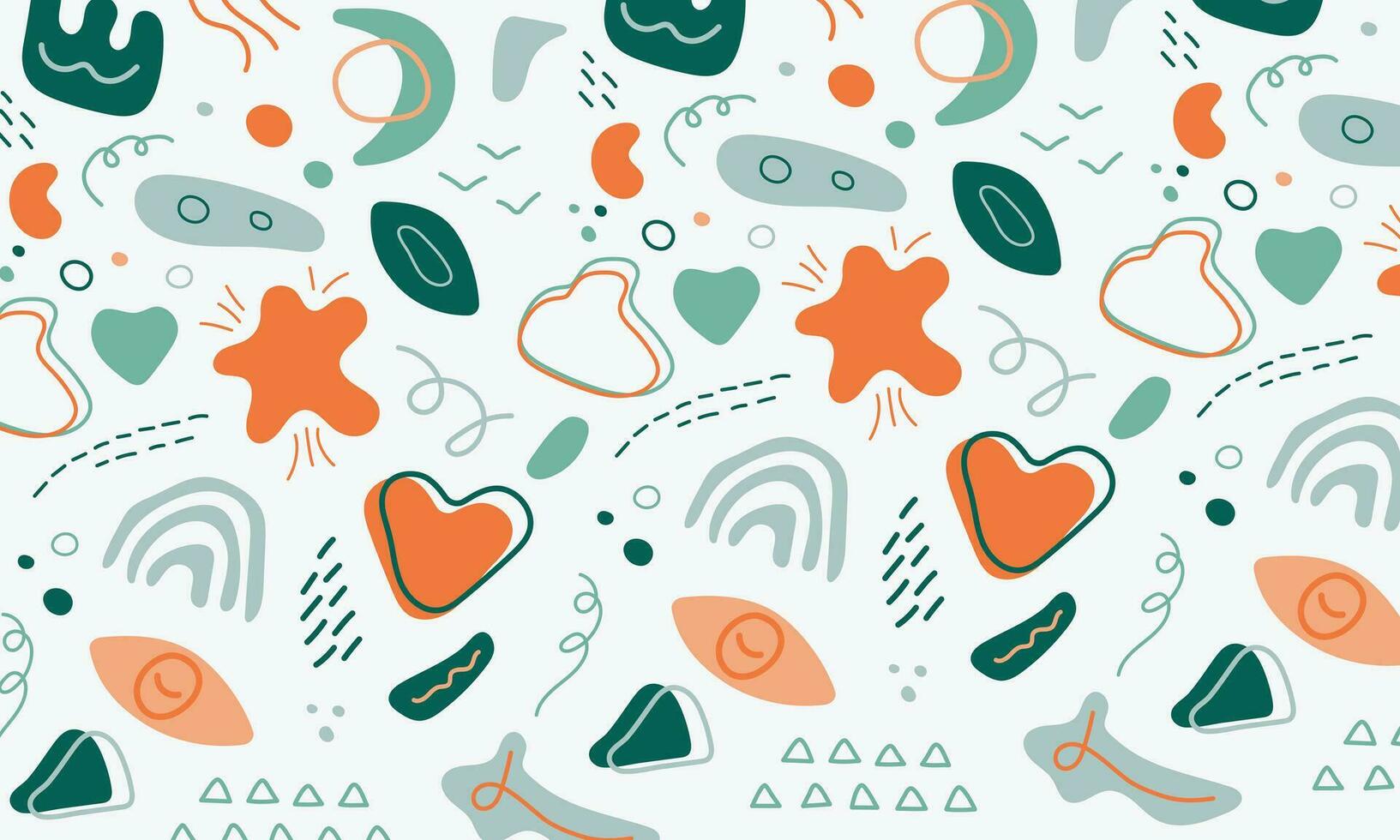The illustration features a whitish-light greenish background adorned with various abstract shapes and patterns, reminiscent of wallpaper or gift wrapping. The primary elements include orange objects such as hearts with green outlines, stars, and other starfish or jellyfish-like forms. Curved orange globs and green crescent moons add to the eclectic mix. Green shapes are prevalent, with triangles arranged in rows, green hearts, football-like ovals with circular centers, dots, and squiggly lines weaving throughout the design. Swirls of green and blue, as well as green circles and dots, contribute to the overall abstract composition. The image showcases a repeating pattern with these whimsical, abstract shapes, creating a playful yet nondescript graphic array.